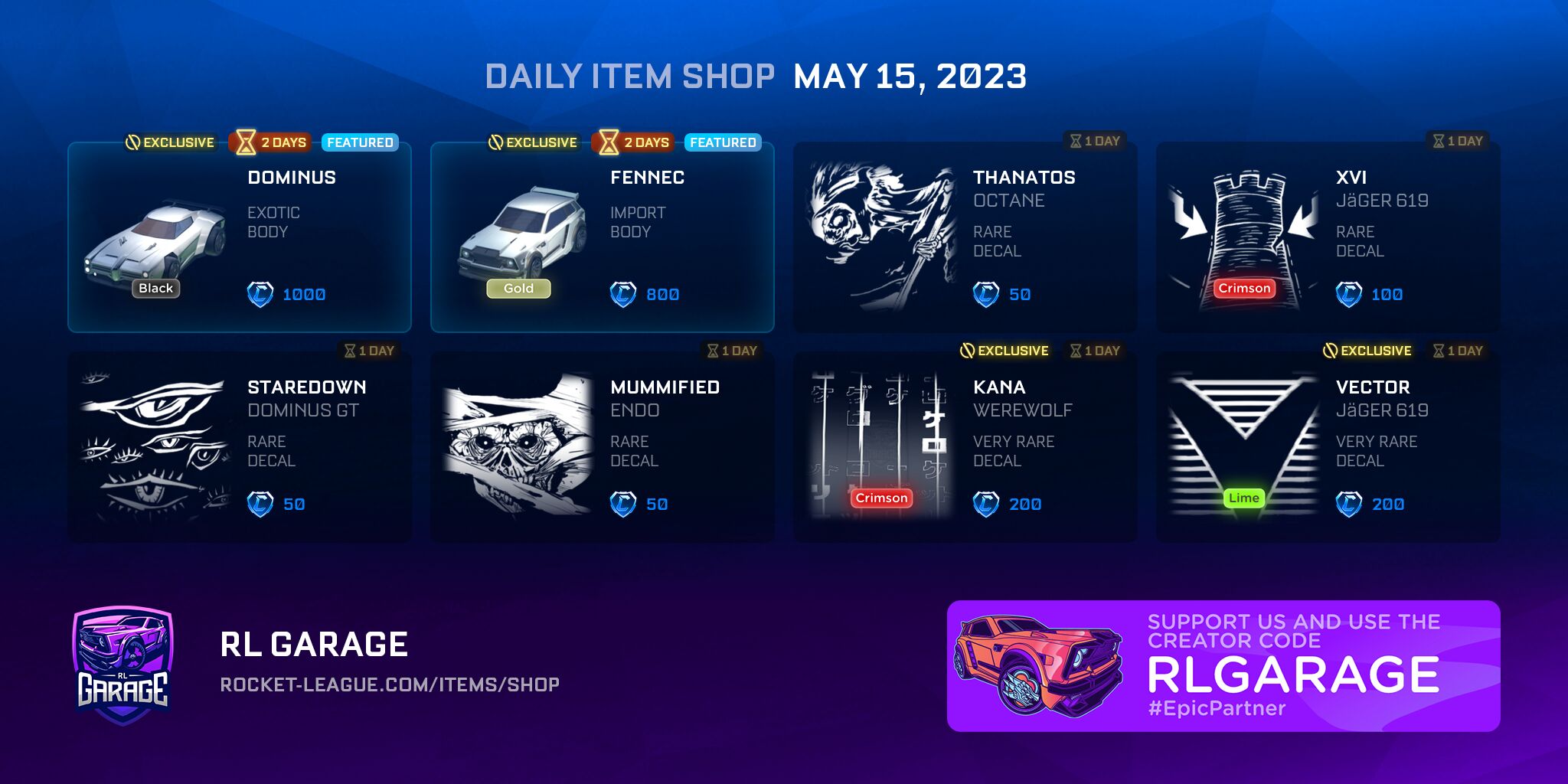This image is a digital screenshot from the popular game Rocket League, showcasing the in-game garage where players can upgrade their vehicles by adding new items. The background features a gradient that transitions from blue at the top to purple at the bottom. At the very top of the screenshot, there's a title that reads "Daily Item Shop May 15, 2023."

Below the title, there are four boxes displaying available items for purchase. The first two boxes feature cars: the Dominus Exotic Body in white and the Fennec Import Body, also in white. The next two boxes showcase logos representing decals that players can apply to their cars: the Thanatos Octane Rare Decal and the XVI Jaeger 619 Rare Decal.

Further down, there are four more boxes, all containing logos of additional decals. These include the Staredown Dominus GT Rare Decal, the Mummified Endo Rare Decal, the Kana Werewolf Very Rare Decal, and the Vector Jaeger 619 Very Rare Decal.

At the bottom of the screenshot, there is a link to RLGarage (rocket-league.com/item/shop), suggesting these items can be browsed or purchased through the Rocket League Garage. A note encourages users to support creators by using the creator code RLGarage, identified as an epic partner, indicating a form of in-game advertisement for item purchases.